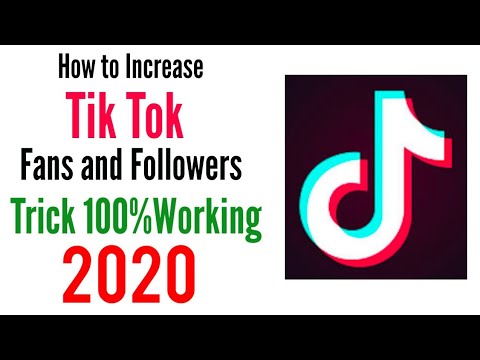"Digital advertisement with a central message in black, red, and green text on a white background flanked by black rectangles on the top and bottom. The text reads:

- In black print: 'How to Increase'
- In red print: 'TikTok'
- In black print: 'Fans and Followers'
- In green print: 'Trick 100% Working'
- In red print at the bottom: '2020'

To the right of the text is the TikTok logo, which is a black square featuring a stylized musical note in teal, white, and red. The phrases 'How to Increase' and 'Fans and Followers' utilize capital H, I, F, and other important words are capitalized for emphasis. The word 'TikTok' is written as 'TIKTOK' in red, and 'Trick 100% Working' has capital T and W."